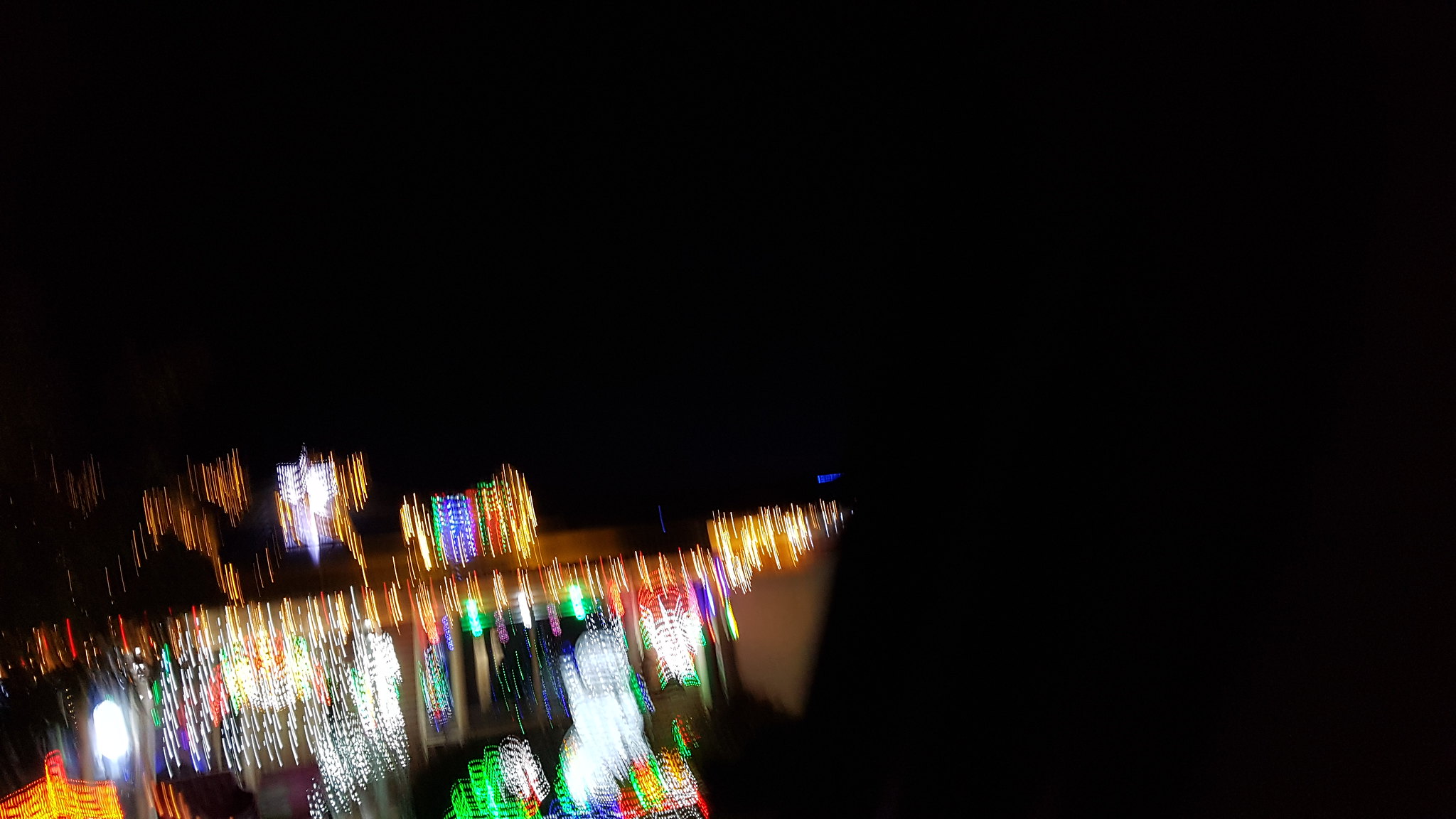This nighttime photograph, captured in landscape format, is predominantly shrouded in darkness, with roughly 75% of the image enveloped in blackness. The lower left quarter of the image, however, is alive with an array of blurred lights, suggesting rapid movement or an unsteady hand during the capture. A kaleidoscope of colors emerges amidst the blur, with hues ranging from white, yellow, and orange to blue, purple, and red. These colors appear in various undefined shapes. There is a notable section featuring a vibrant concentration of yellow, blue, purple, red, yellow, and white lights clustered together. 

One distinctive element is a dead-straight row of lights situated above an assortment of white lights and set against a backdrop washed with green, pink, purple, yellow, and white illumination. 

In the foreground, near the center of the image, are two prominent sections of light: one predominantly green and the other primarily red. An expansive patch of orange light dominates the bottom left-hand corner. The exact nature of the scene is ambiguous; it could be an urban street drenched in nightlife, the interior brilliance of a casino, or another vibrant venue. The photo, a symphony of blurred luminance, leaves the details open to interpretation.